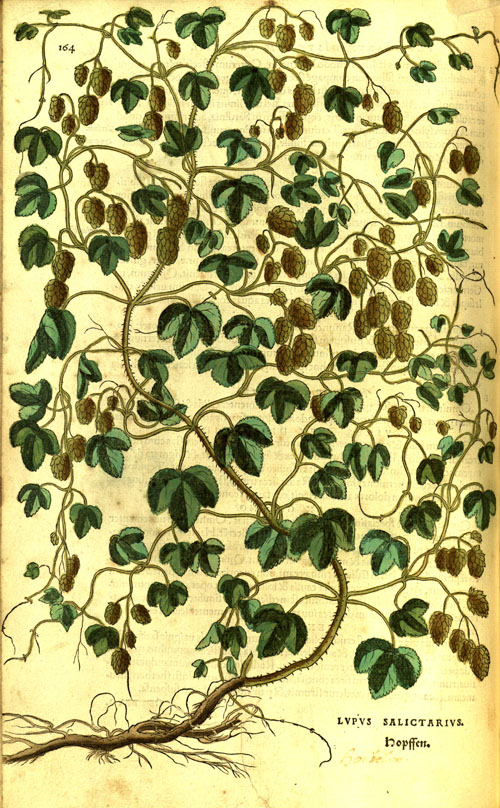The image depicts a meticulously drawn plant with a prominent root system extending upward into spiky branches that further subdivide into smaller branches. These branches bear heavy, green leaves and small, pine-cone-like pods, resembling a vine plant. The page appears weathered and yellowed, suggestive of age, with evident darkening along the right edge. The illustration is very crisp despite the worn-out page, which likely comes from an old book, indicated by the number 164 in the upper left corner. At the bottom, some writing is present including "LVPVS, Salictarvis" and possibly a foreign word "noptfen." This precise and detailed drawing might be categorizing a specific plant, possibly hops given the pod-like structures, though some interpretations suggest a grapevine due to the fruit-like berries depicted.